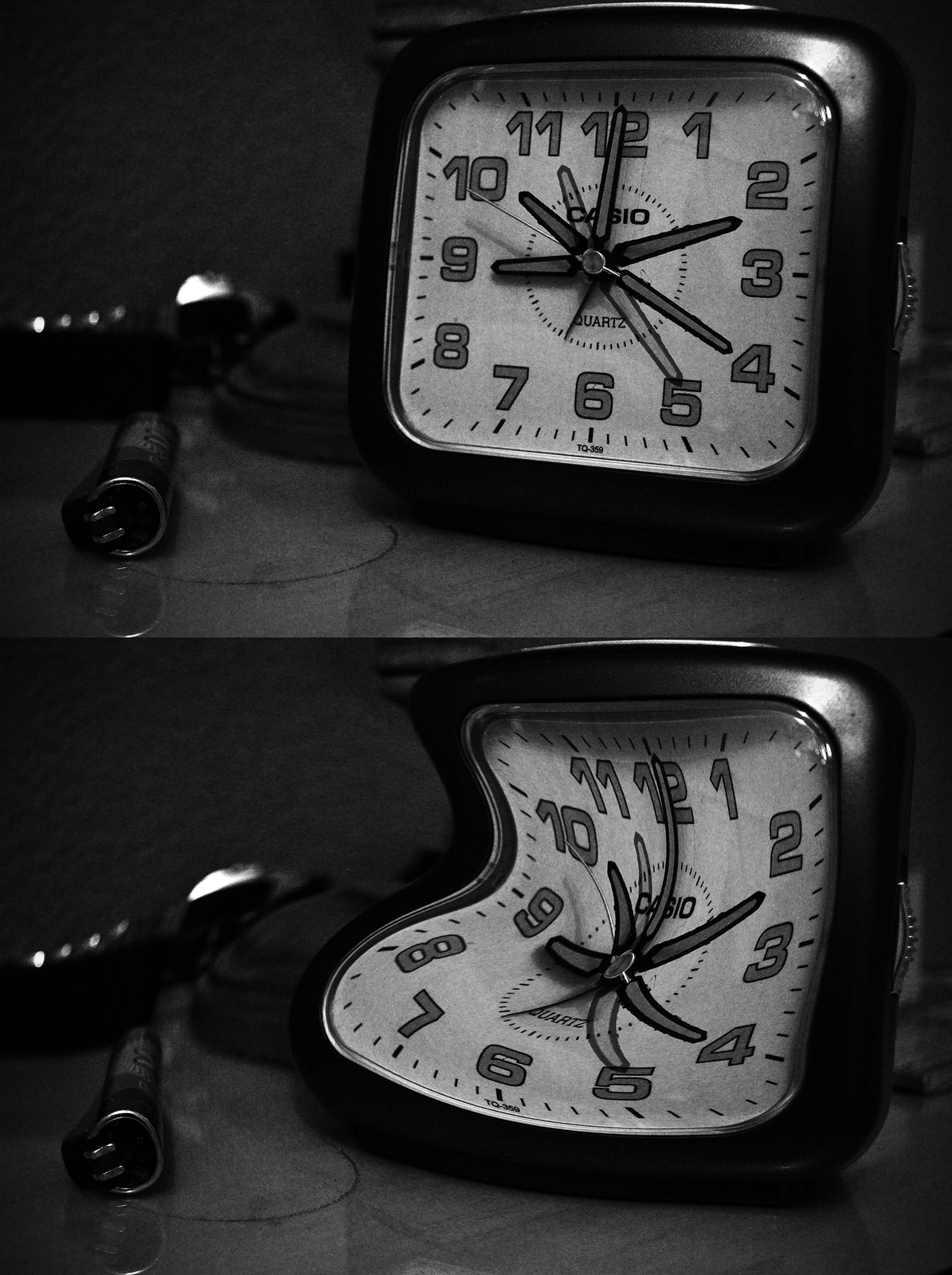The image consists of two distinct photos of the same clock, arranged one above the other. 

In the top photo, the clock is placed on a desk along with various metal objects. The image is in black and white, rendering all colors indistinguishable. The clock itself is square, with a white face and darker numerals. Several hands populate the face: 
- One hand points directly at the 12.
- A darker minute hand also points at the 12.
- An hour hand, not as dark, points at the 11.
- Another darker hour hand indicates the 10.
- A similarly shaded hour hand points to the 9.
- Additionally, a darker minute hand shows 12 minutes.
- Light minute hands point to the 4 and 5.

In the bottom photo, the same clock is represented but appears twisted and distorted, as if viewed through a watery lens or during a hallucination.